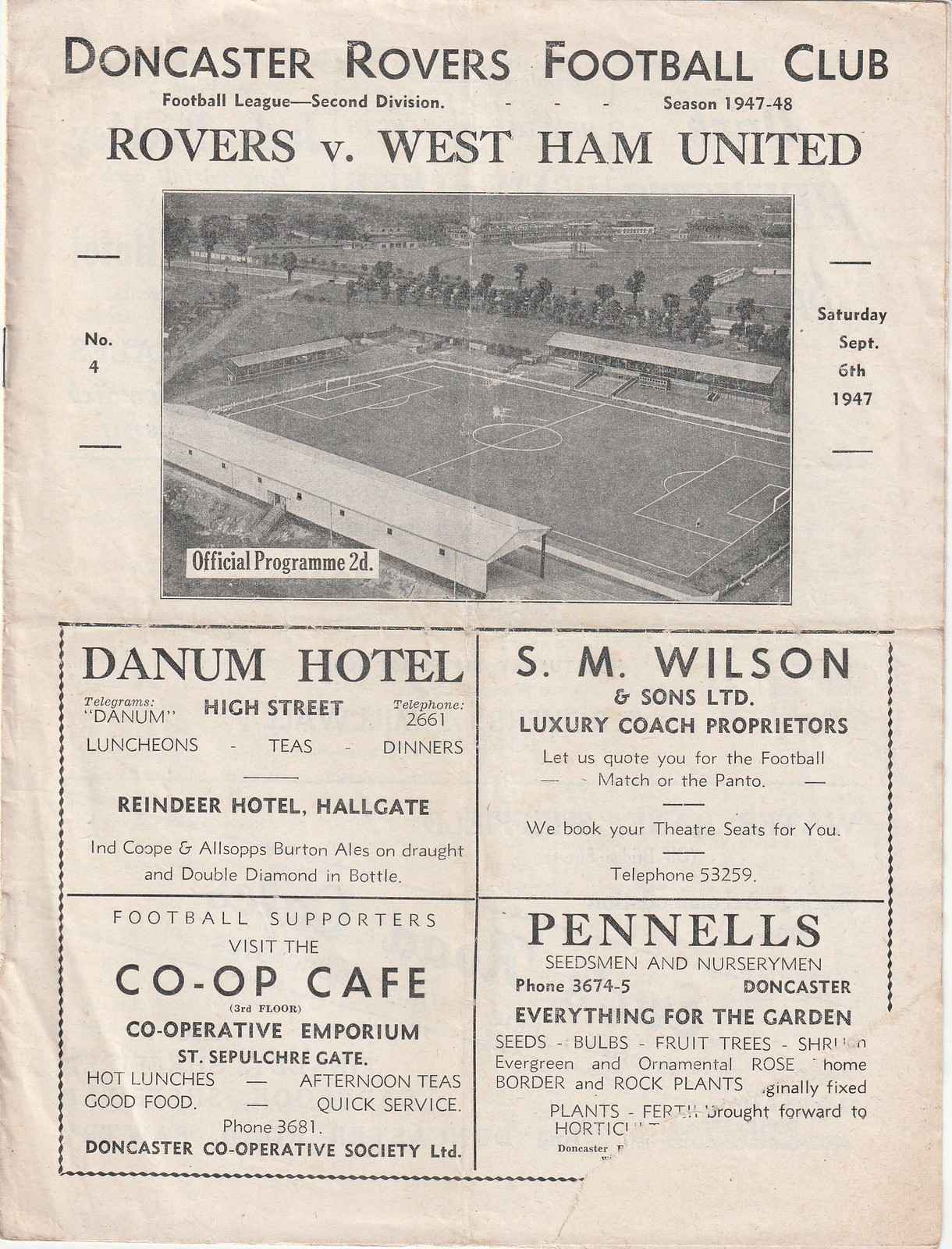This is an aged, beige-hued sports program for a football match between Doncaster Rovers Football Club and West Ham United, dated September 6, 1947. The program, likely from London, England, features "Doncaster Rovers Football Club" prominently in black text at the top. Beneath this header, the match details "Rovers vs. West Ham United" are bolded, and to the right, the date and weekday "Saturday, September 6, 1947" are noted. Centrally positioned on the page is a black-and-white photograph of a football field, flanked by the number '4' on one side and the word 'Saturday' on the other. Beneath the photograph, the page is divided into four advertisement boxes. The top left advertises Danum Hotel, the top right features S.M. Wilson, the bottom left corner promotes Co-op Cafe, and the bottom right ad, partially obscured due to a tear, likely represents Pennells. This rip exposes writing from the subsequent page underneath. The program bears evidence of water stains, a central fold, and fringes of wear, visibly highlighting its vintage nature.